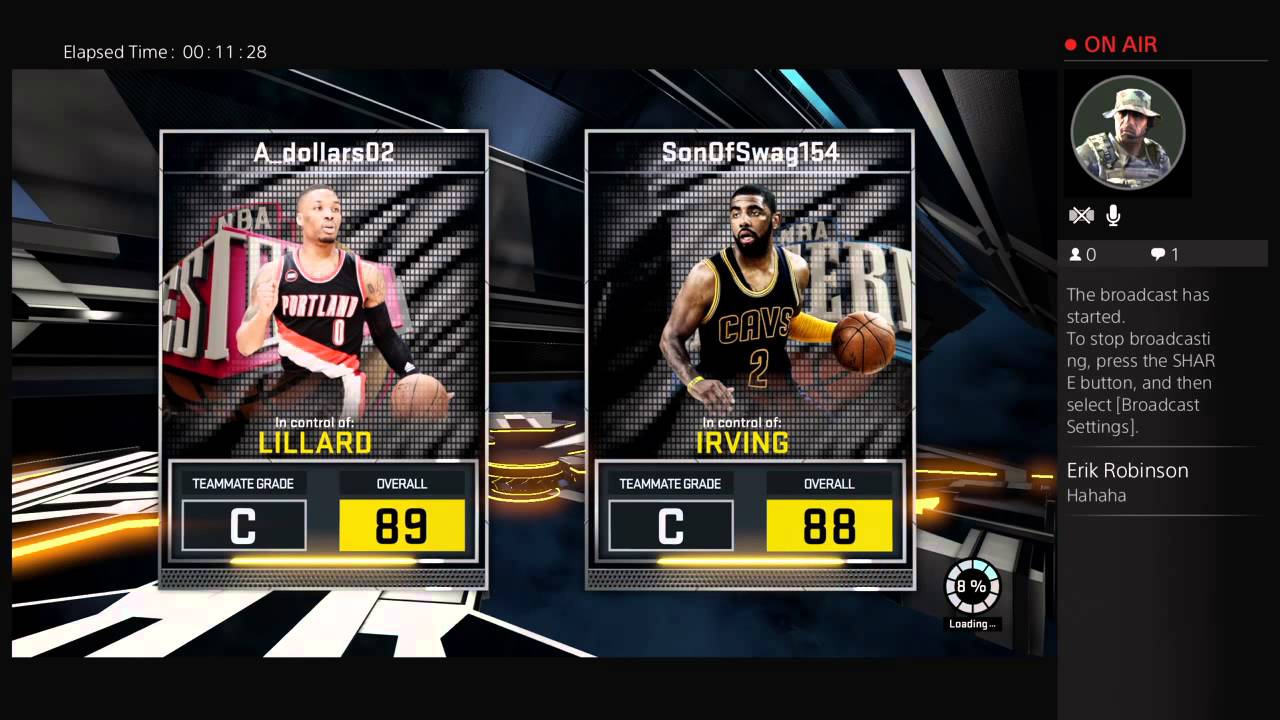This screen capture from a video game depicts an interface with various elements indicating player details and broadcasting status. The top left corner displays a lap time of 11 minutes and 28 seconds. Below this, two rectangles show the profiles of professional basketball players. On the left, the player named "Lennard" is highlighted, with text indicating control by user "A_DOLLARS02." An African American player wearing a black Portland Trail Blazers jersey with the number 0 is seen holding a basketball and looking to the right. His performance is noted with a "Teammate Grade" of C, displayed in a bold black square with a white border, and an "Overall" rating of 89 in a yellow rectangle.

On the right-hand side, the profile of another player, Kyrie Irving, is shown, controlled by user "SonOfSWAG154." This player has a "Teammate Grade" of C and an "Overall" rating of 88. A red "On Air" indicator on the right highlights an active broadcast, accompanied by various interface elements, including the profile picture of a military character in green gear, a speaker icon with an X (indicating it is off), a microphone, a silhouette icon with the number zero, and a comment bubble with the number one.

The broadcast details in gray text instruct that "The broadcast has started. To stop broadcasting, press the SHARE button, and then select [Broadcast Settings]." Bold white text at the bottom reads "Eric Robinson," followed by the comment "hahahaha" in gray.